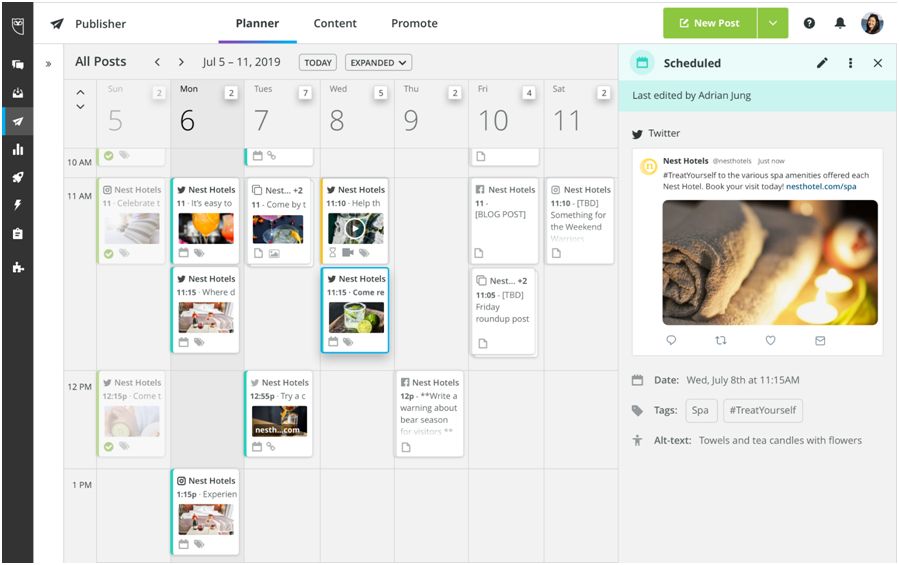The image, featured on a publishing website, includes a thin vertical black bar on the left side that runs the entire length of the image. This bar showcases white symbols including a graph icon, a male symbol, a rocket ship, a lightning bolt, and what appears to be a notepad or clipboard symbol. 

To the right of this black bar, at the top of the image, there is a horizontal white bar displaying the website's name, "Publisher," accompanied by a paper plane logo. Alongside this header, there are tabs labeled "Planner," "Content," and "Promote," each with "New Post" buttons situated on the right. Additionally, the top right corner features a help button, a notification symbol, and a user profile icon.

Below the white header bar, the background shifts to a light gray, showcasing a calendar interface. This calendar currently displays posts scheduled for the week of July 5th through July 11th, 2019. Each day within this date range includes various images and detailed scheduling information for planned posts and activities.